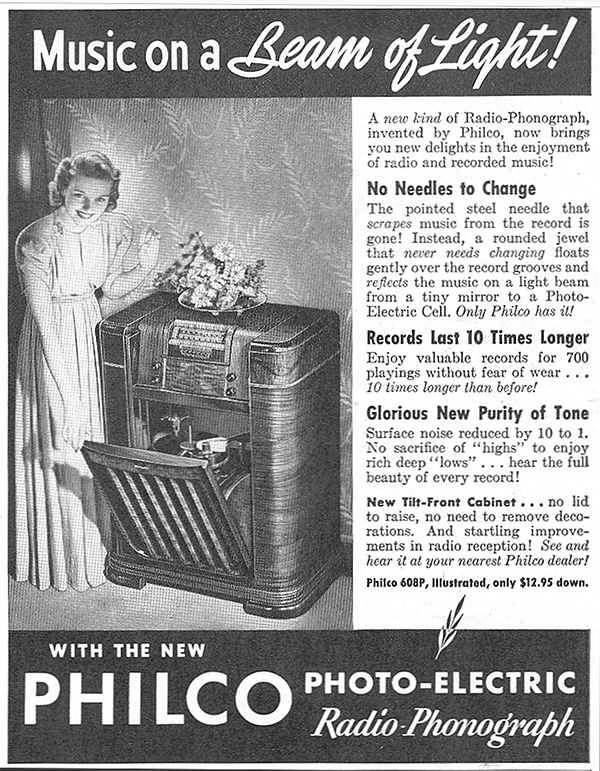This vintage black-and-white newspaper advertisement prominently features the headline, "Music on a Beam of Light." The ad is for the new Philco Photoelectric Radiophonograph, which is a multifunctional piece designed like a bookcase. At the top of the wooden box is a radio, and at the bottom, accessible via an oven-like door, is the record player. 

The central image displays a woman in a floor-length dress, smiling as she stands beside the open radiophonograph, with a record visible on the player. The top surface of the player is adorned with a decorative plate of flowers. 

The right side of the advertisement details the revolutionary features of the Philco device, emphasizing that it requires no needle changes, resulting in records lasting ten times longer. Instead of a needle, a rounded jewel that never needs changing gently floats over the record grooves, reflecting music on a light beam from a tiny mirror to a photoelectric cell, an innovation unique to Philco. This results in substantially reduced surface noise and no loss of either high or low frequencies, allowing the full beauty of every record to be heard. 

The ad also highlights the new tilt front cabinet design, which eliminates the need to raise a lid or remove decorations to access the player. Additionally, it boasts improved radio reception. The model featured in the illustration is the Philco 608P, available for $12.95 down at Philco dealers.